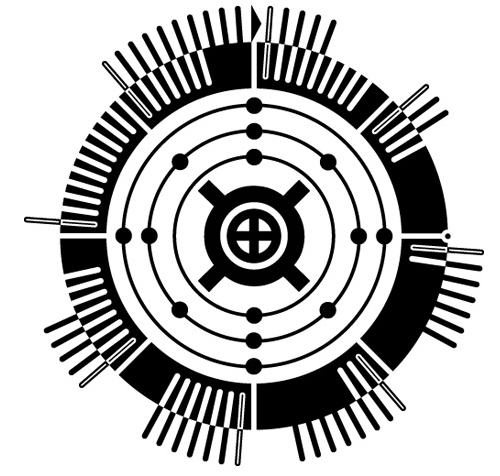This highly detailed black and white illustration resembles a complex emblem or target, potentially a puzzle, maze, or game. The design prominently features concentric circles and intricate patterns. At the center lies a black cross or plus sign enclosed within a black circle. Surrounding this is a white border, followed by a black circle with four points extending outward. This pattern continues with additional black circles, each interspersed with small black-filled circles or 'balls' along their paths. The outermost ring is notably thicker, decorated with white lines, some of which are partially black-filled. An arrow, comprising a thin pointer, is positioned at the top of the image, directing to the right. Overall, the emblem includes components like multiple layers of circles, a central cross, equidistant stubs or pointers, and numerous small round elements, all meticulously arranged in a harmonious yet complex structure.